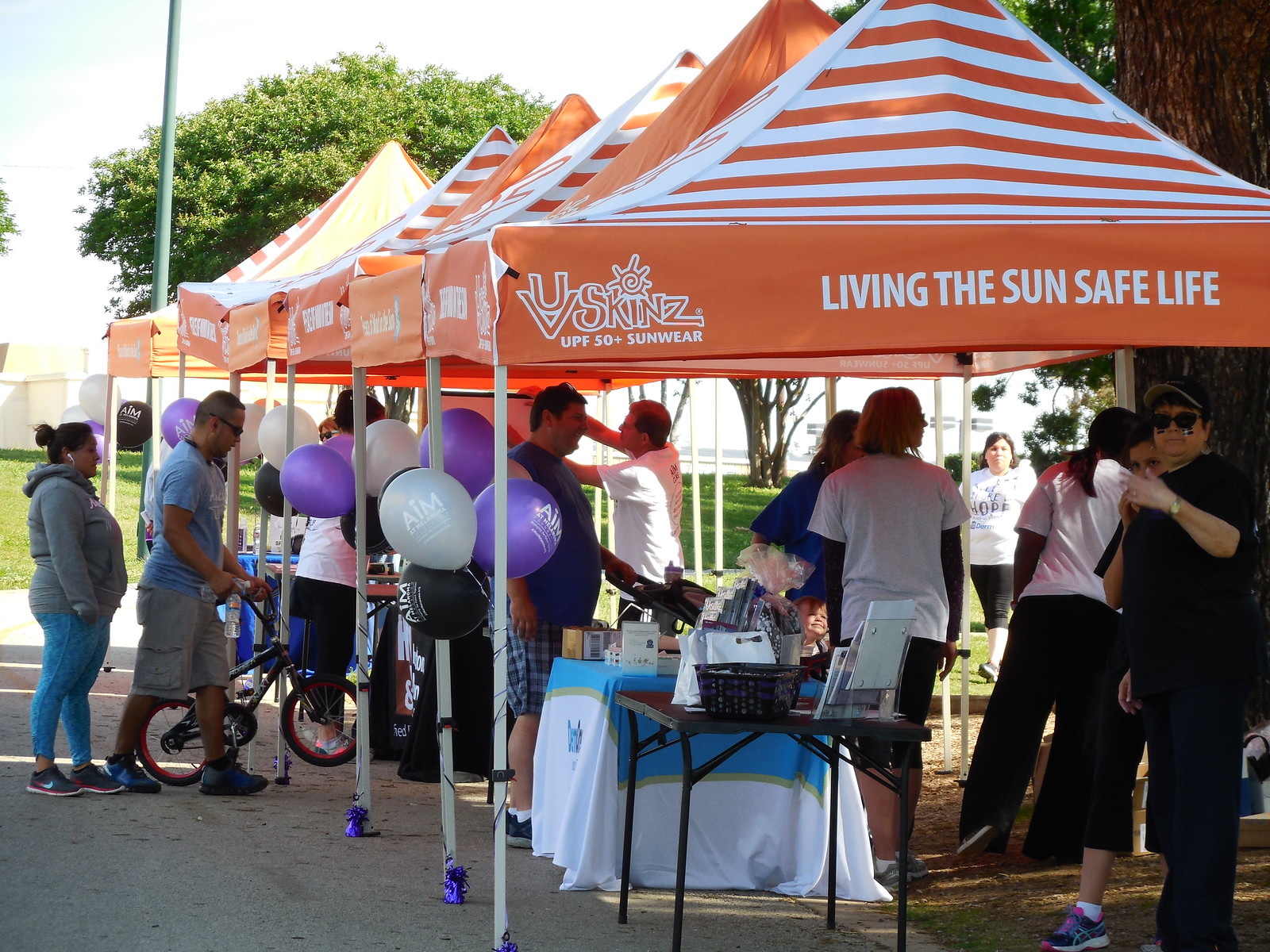The image captures a bright outdoor event set up in a parking lot, featuring a row of orange tents with alternating white and orange striped canopies, supported by white poles. The tents, primarily providing shade, convey messages in white letters such as "Living the Sun Safe Life" and "UPF 50+ Sunwear, SKINZ," accompanied by a sun graphic. The ground beneath is a mix of concrete and patchy grass. 

Attendees, dressed casually in shorts and hoodies, wander among various booths, exploring items and brochures displayed on tables. The first booth features a blue and white tablecloth, with signs and products arranged neatly. Purple, silver, and black balloons with the letters "AIM" tied to tent poles suggest either the event's name or a sponsor. One particular highlight is a man on the right, wearing sunglasses and giving a thumbs up, while another man on the left carries a small child's bike. The setting is lively, with people mingling and engaging with the displays against a backdrop of trees and a bright, blue sky.